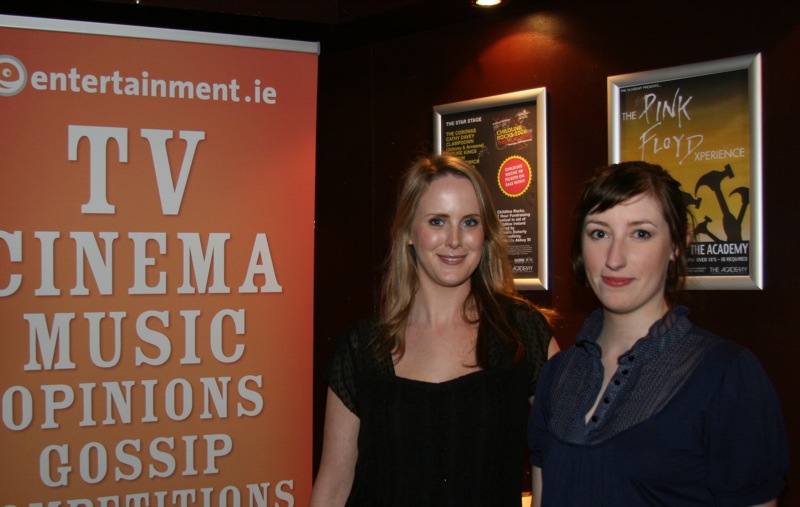In the image, two well-dressed women stand side by side in the bottom right corner, facing the camera with smiles. The woman on the left has long blonde hair and wears a black top with short sleeves, while the woman on the right has brunette hair pulled back and is dressed in a dark blue top with a lacy collar. Behind them, two posters adorn the wall in the upper right corner, while to the left of the women, a large orange sign prominently reads "Entertainment.ie" followed by "TV, Cinema, Music, Opinions, Gossip" in center-aligned text. The scene, likely indoors and potentially set in a movie theater, features a varied color palette including black, tan, dark blue, yellow, red, orange, and gray.